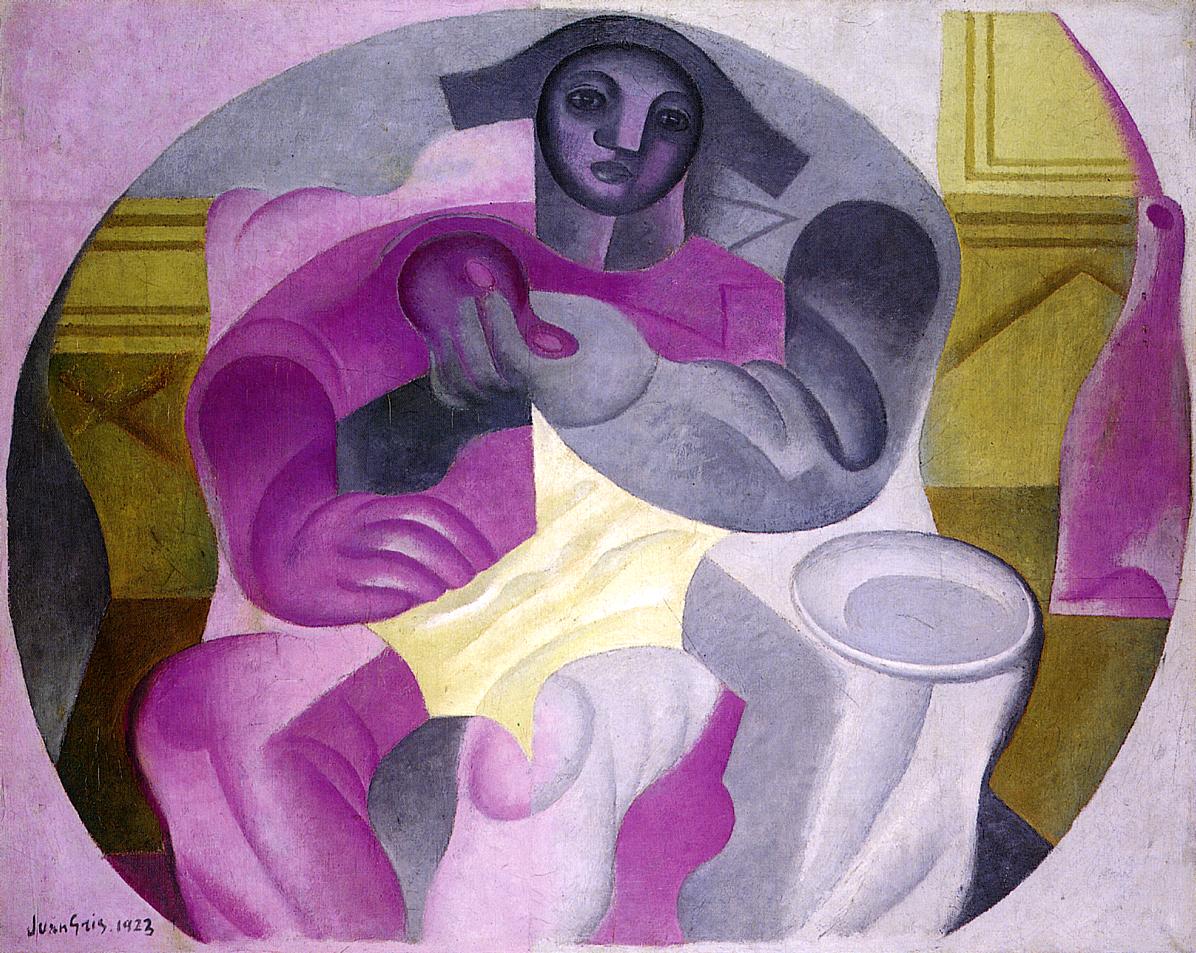The painting depicts an abstract, modern art style image primarily in shades of gray, purple, and pink. The central figure appears to be a heavy, round woman with a disproportionately small head compared to her large arms and legs. She is seated, perhaps on a chair, with one leg bent, and a white plate rests on her left knee. The woman wears a combination of light purple and pink clothing, with one leg clad in white. Her face features a mix of black, white, and gray. In one hand, she appears to be holding an undefined object that vaguely resembles the head of a purple duck. The background includes a greenish-beige wall and a yellow table, with what looks like a wine bottle on it, hinting at a living room setting. The image composition is soft and overlapping, layering various colors and shapes to create a harmonious yet complex visual. At the bottom left corner, the painting is signed with the name "Juan" and dated 1923.